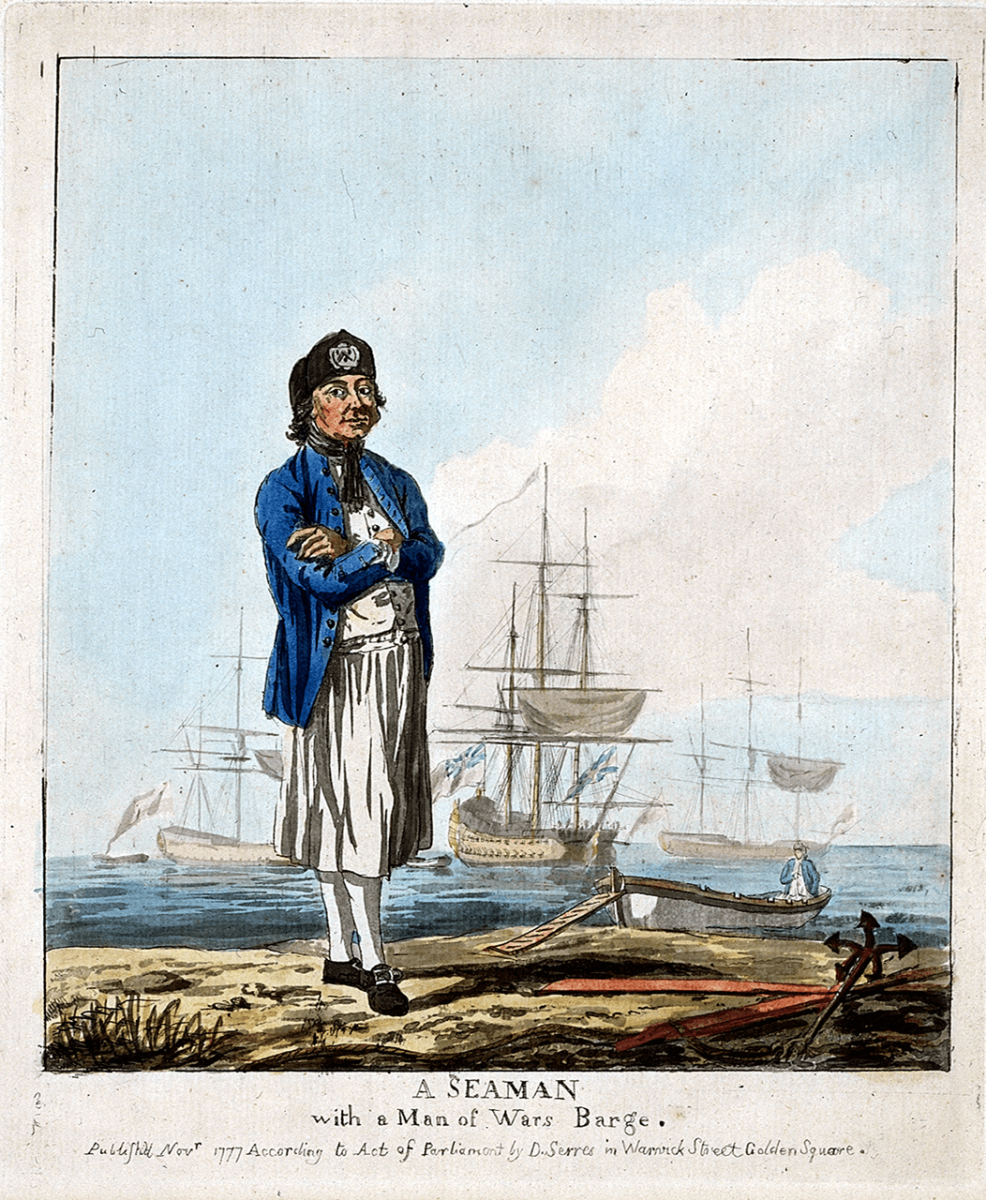This detailed watercolor painting, set against an aged, light gray textured paper, portrays a seaman standing resolutely on a brown shore. The seaman is attired in a distinctive blue coat with a blue overcoat, white baggy trousers or lower, white leggings, and brown buckle shoes. His dark black beret or cap complements his folded arms, which suggest a stolid demeanor.

Behind him, the scene unveils a tranquil blue ocean where three large wooden sailboats, their sails neatly furled, rest in the bay. One of these is a man-of-war, marked by double rows of cannon ports, flanked by two other sailboats devoid of visible cannons. Closer to the shore, a smaller rowing boat with another man seated at the back has recently arrived.

Above the sailor and the vessels, a serene sky with white clouds stretches out, enhancing the nautical theme. Below the painting, a caption reads, "A Seaman with a Man of War's Barge, published November 1777 according to Act of Parliament by D. Saraz in Warwick Street, Golden Square." This inscription, written in black, provides historical context and authenticity to the image.